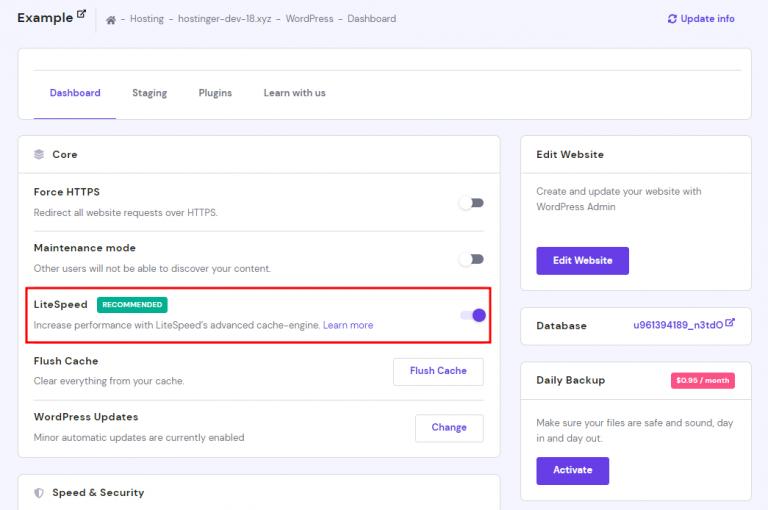The image is of a web hosting dashboard, specifically for managing a WordPress website. At the top right corner, there is a clockwise circular arrows icon representing the update information. The main tabs at the top include "Dashboard", which is the current view, "Staging", and "Plugins".

Below the main tabs, there is a white box labeled "core" in black text. Beneath that, another white box features the "Force HTTPS" setting, which redirects all website requests over HTTP; this feature is currently toggled off. Additionally, there is a "Maintenance Mode" setting, which is also turned off.

Highlighted in red is the "LiteSpeed" section, which promotes the use of LiteSpeed's advanced cache engine to enhance performance. This section includes more information and an option to turn it on. Adjacent to it is the "Flush Cache" button, used to clear everything from the cache.

The "WordPress Updates" section indicates that minor automatic updates are currently enabled, with an option to change this setting. Below this is the "Speed and Security" section, leading to the "Edit Website" button for creating and updating the website through WordPress admin.

Further down, there is a "Database" section followed by an option for "Daily Backup" services for 95 cents a month. The accompanying message reads, "Make sure your files are safe and sound day in and day out." There is also a purple button labeled "Activate" for enabling the daily backup service.